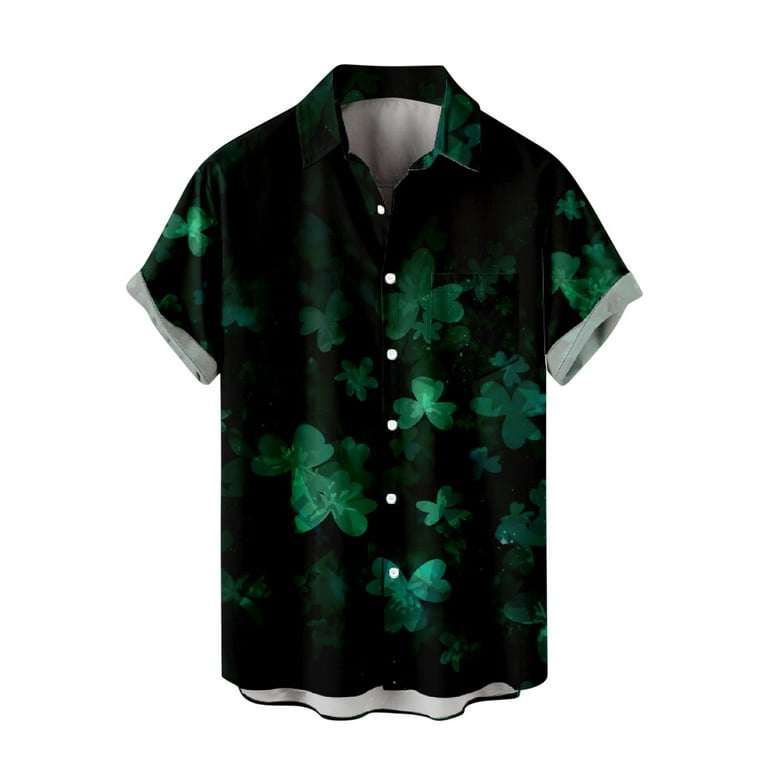This image showcases a St. Patrick's Day-themed short-sleeve button-up shirt, prominently featuring a black exterior adorned with vibrant green clover leaves. The shirt, crafted from what appears to be soft cotton material, is distinguished by its black background contrasted by the bright, almost glowing centers of the green three-leaf clovers. The buttons running down the front are white, with all but the top two fastened, contributing to its casual yet polished look. The sleeves are slightly rolled up, revealing white cuffs, echoing the shirt's white inner lining. Additionally, a hint of light bluish-green cloth peeks out near the sleeve edges, adding a subtle touch of contrast. This product image, presented vertically as if on a clothing website, provides a clear view of both the black and green patterned external fabric, and the stark white interior, encapsulating the spirit of festive wear for St. Patrick's Day.